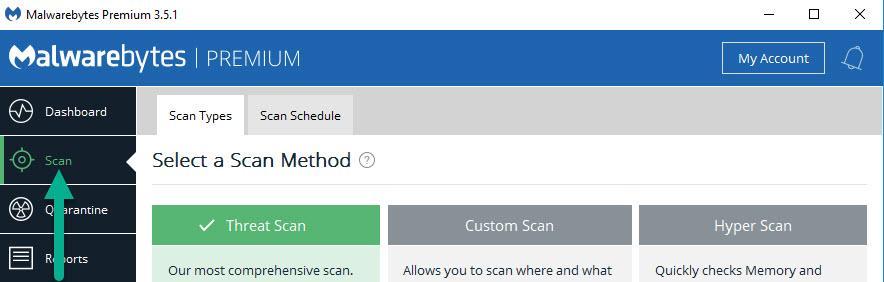The top portion of the screen features a blue malware symbol with devil horns, indicating the application Malwarebytes Premium version 3.5.1. Adjacent to this are the window control buttons: minimize (hyphen), maximize (square), and close (X). Beneath this section is a medium blue banner displaying 'Malwarebytes,' where the 'M' doubles as the malware symbol and is more pronounced, while 'bytes' and 'premium' are presented in a lighter font. To the right of the banner are buttons for 'My Account' and a notification bell.

Along the left side of the interface is a vertical black menu with clickable options: 'Dashboard,' 'Scan,' 'Quarantine,' and 'Reports,' each accompanied by respective icons. A green arrow highlights the 'Scan' option, which is currently active on the main screen. This panel is gray and displays options for 'Scan Types' and 'Scan Schedule.' The selected view under 'Scan Types' allows users to choose their scan method. The available choices are 'Threat Scan,' 'Custom Scan,' and 'Hyper Scan,' with 'Threat Scan' being the currently selected option.